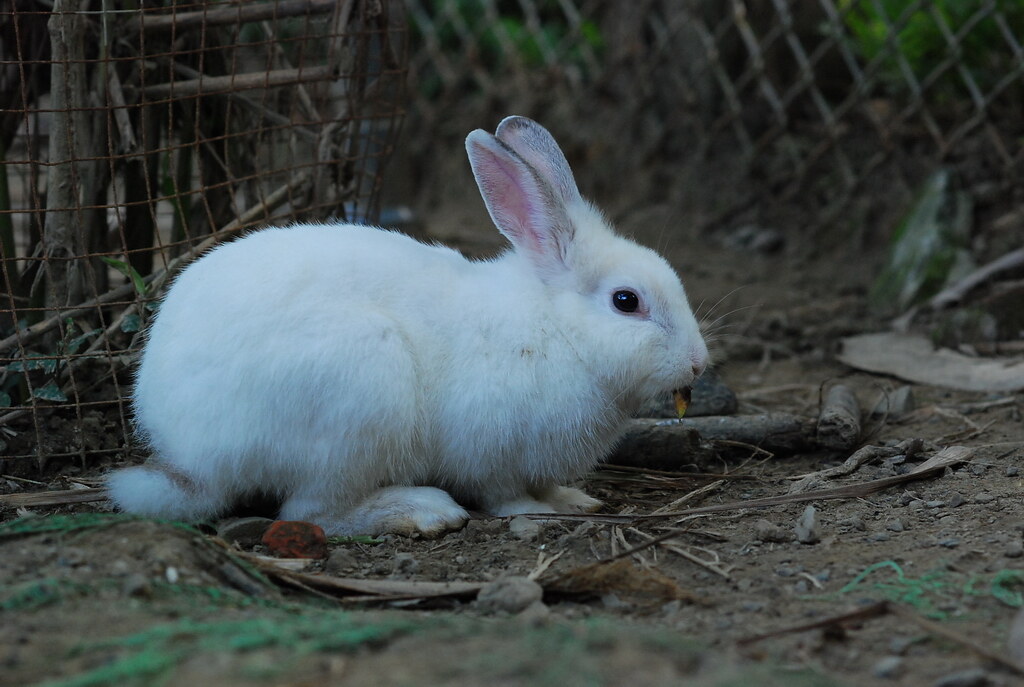This is a close-up photo of a white bunny with pink and slightly gray ears, captured outdoors. The bunny is in a side profile, showing one of its black eyes and its pink nose. It appears to be munching on a leaf. Surrounding the bunny is a mix of dirt, twigs, and dried leaves, with a hint of green moss visible. In the background, there's a wire structure that could be part of a cage or a yard fence, making it unclear whether the bunny is a pet or a wild one in a fenced garden. The bunny's compact body is resting on all fours, giving it an adorable and inquisitive appearance.